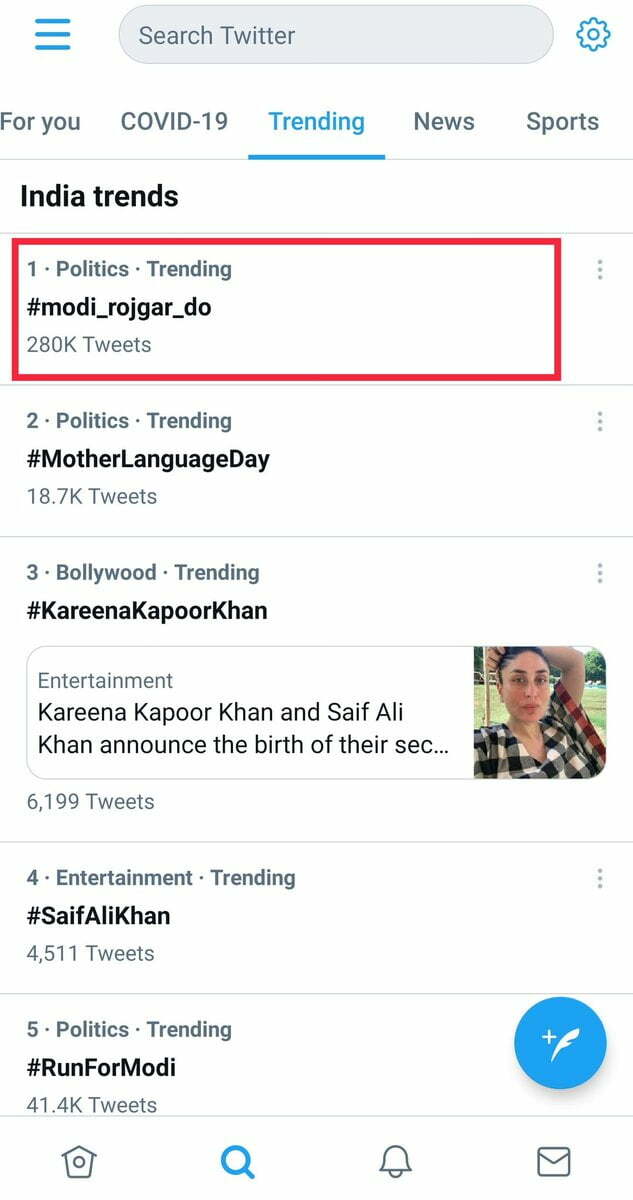**Detailed Caption:**

This is a screenshot taken from a tablet or smartphone displaying a Twitter trending page. The top bezel features three cyan blue lines. Below this, an oval search bar, mid-gray in color with black text that reads "Search Twitter," is positioned. Adjacent to the search bar on the right side is a cyan blue gear icon.

At the top of the screen, dark gray tabs labeled "For you" and "COVID-19" are visible. The "Trending" tab is selected, highlighted in cyan blue with a cyan blue underline. Within this section, categories such as "News" and "Sports" are shown in gray.

Below these tabs, there is a white background area showcasing "India Trends" in bold black text, followed by a thin separator line. The first trending topic is displayed within a red rectangle indicating "1. Politics · Trending," followed by the trending hashtag "#MODI_ROJGAR_DO" in bold black text. Below this, "280K Tweets" is noted in dark gray font.

The second trending topic is outlined in another rectangle, featuring the numeral "2" and "Politics · Trending." The hashtag "#MotherLanguageDay" is in bold black text, showing "18,000 Tweets" underneath.

The third trending topic, "3. Bollywood · Trending," highlights the hashtag "#KAREENA_KAPOOR_KHAN" in bold black. A corresponding image shows a woman in a white and black plaid shirt with her hand over her head. The text further explains that Kareena Kapoor-Khan and Saif Ali Khan announced the birth of their second child, but the full description is cut off and ends with an ellipsis. This item has "6,199 Tweets."

For the fourth trending topic, labeled as "4. Entertainment · Trending," the hashtag "#SAIF_ALI_KHAN" appears in bold black, accompanied by "4,511 Tweets" in gray.

The fifth topic is under "Politics · Trending," showing the hashtag "#RunForModi" in bold black text and highlighting "41.4K Tweets." Additionally, a dark blue circle with a white plus sign and a white feather icon is present underneath.